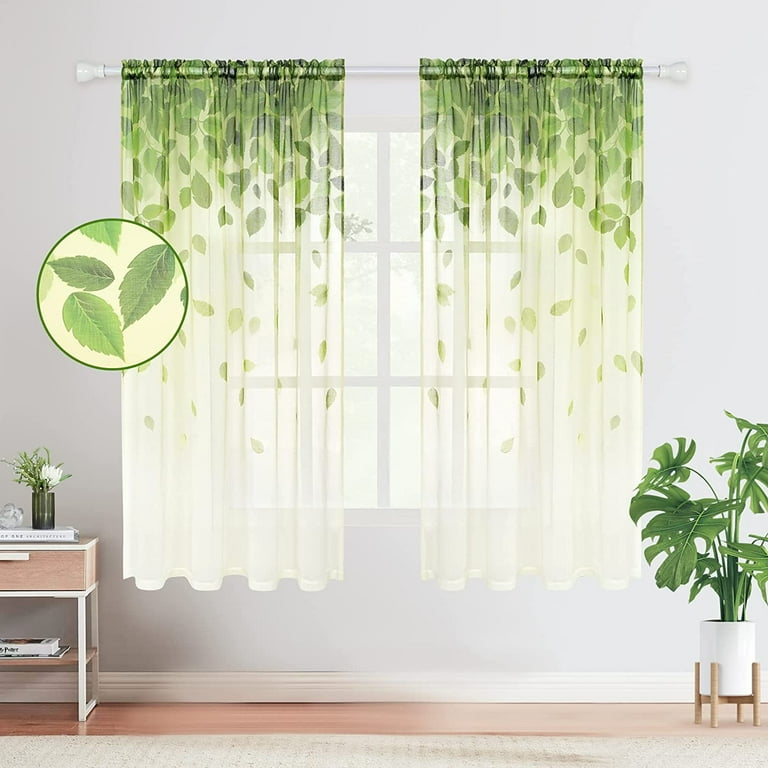The photo captures a serene room featuring a prominent window with two sheer white curtains adorned with a vivid green leaf design that intensifies towards the top and gradually dissipates, leaving the bottom third completely white. Centered above the window is a white horizontal curtain rod. The left side of the window shows a detailed circular magnified graphic of the leaves, emphasizing their vibrant design. Below this visual focal point, an end table with a shelf and a drawer holds a vase containing a single flower, an alarm clock, and books. To the right of the window, a white planter houses a tall greenhouse plant. The backdrop is a white-greyish wall, and a light-colored rug lies on the floor, completing the tranquil atmosphere of the room.